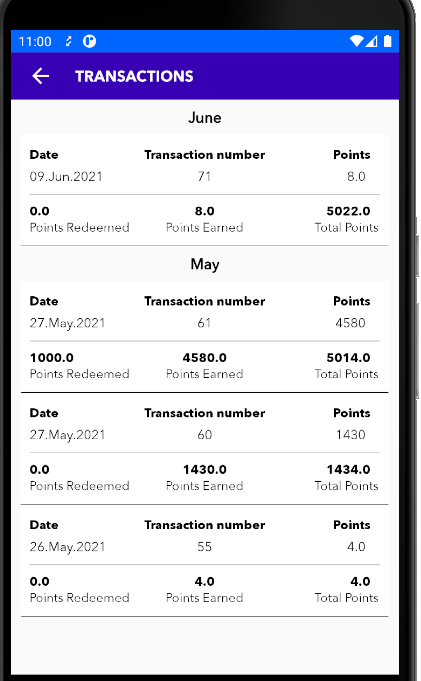This screen capture depicts a financial application interface on what appears to be a tablet, likely due to its shape. The interface shows a status bar at the top displaying the time "11:00," alongside icons including a data transfer symbol and another icon resembling an eye with the dot positioned to its right. In the top-right corner of the screen, Wi-Fi connectivity, service status, and battery power indicators are visible.

Below the status bar, the screen is divided into sections. The header section is light blue, and immediately below it, a dark blue bar has the heading "Transactions." Under this heading, the interface presents columns labeled "June," "Date," "Transaction Number," and "Points" in black text on a white background.

The records begin with June, listing a single transaction entry under the respective date and details. Following this, three transactions are listed under May, each associated with specific dates, transaction numbers, and the points accrued for each transaction.

Overall, the color scheme is a blend of blues for the headings with black text on a white background for the transactional details, creating a clear and organized financial summary.